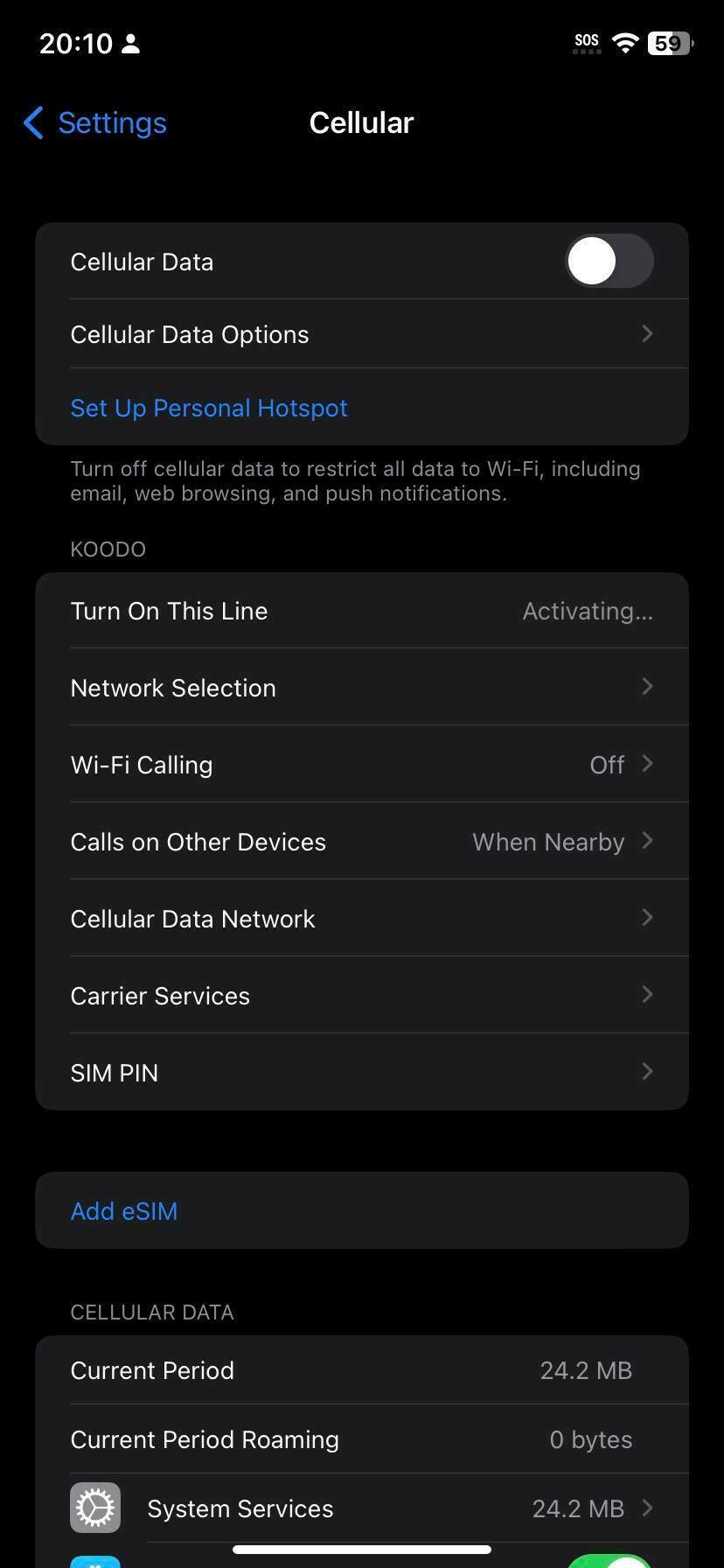The image captures a smartphone screen with a black background. At the top left, the clock displays the time as 20:10 in white text. On the top right, there are various status indicators, including a Wi-Fi signal icon and a battery indicator showing 59% remaining.

Below the status bar, the screen is divided into multiple sections of settings related to cellular options. The first section has a blue heading labeled "Settings" on the left side and the word "Cellular" in white at the center. 

Under the primary heading, there are grouped subsections:

1. **Cellular Data**:
   - *Cellular Data*: Enabled.
   - *Cellular Data Options*: In white.
   - *Set Up Personal Hotspot*: In blue.

2. **Kudu** (The name of the cellular provider or a custom label):
   - *Turn On This Line*: Shows "Activating".
   - *Network Selection*: Option available.
   - *Wi-Fi Calling*: Currently off.
   - *Calls on Other Devices*: Set to "When Nearby".
   - *Cellular Data Network*: Accessible option.
   - *Carrier Services*: Accessible option.
   - *SIM PIN*: Option available.

3. **eSIM**:
   - *Add eSIM*: Highlighted in blue.

4. **Cellular Data Usage**:
   - *Current Period*: 24.2 MB.
   - *Current Period Roaming*: 0 bytes.
   - *System Services*: 24.2 MB. 

The descriptive details and the organization of settings convey a clear snapshot of the cellular settings currently displayed on the smartphone.